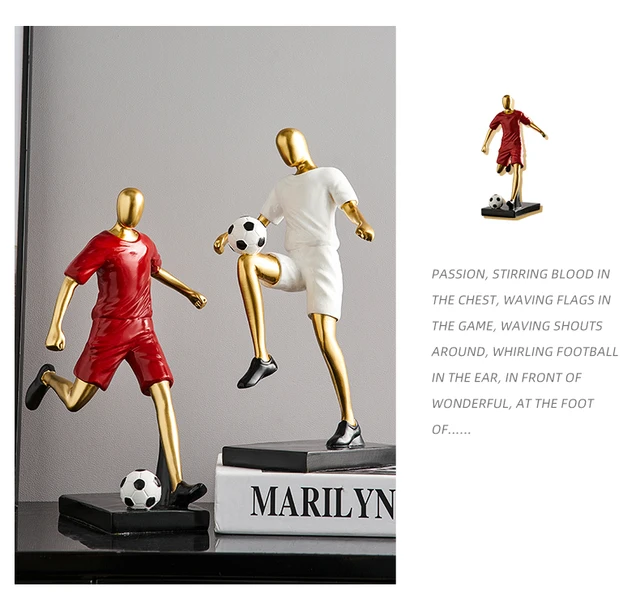This is an image of two golden soccer figurines. Both figurines are placed on a sleek, black tabletop, possibly made of marble or glass, set against a gray painted wall. The figurine on the right is perched on top of a book with a white spine and black letters that read "Maryland." This figurine is wearing a white t-shirt, white shorts, and black sneakers. It is skillfully balancing a soccer ball on its right knee. Meanwhile, the figurine on the left stands on a black square platform and is dynamically posed, wearing a red t-shirt, red shorts, and black shoes. This figure has its right leg pulled back, ready to kick a soccer ball that is on the ground in front of it. Both figurines, notably faceless, exhibit striking action poses with exposed golden limbs. The base of these statues bears an inscription: "Passion stirring blood in the chest, waving flags in the game, waving shots around, whirling football in the air in front of wonderful at the foot of..." This scene captures the enthusiasm and dynamism of soccer through meticulously crafted details.